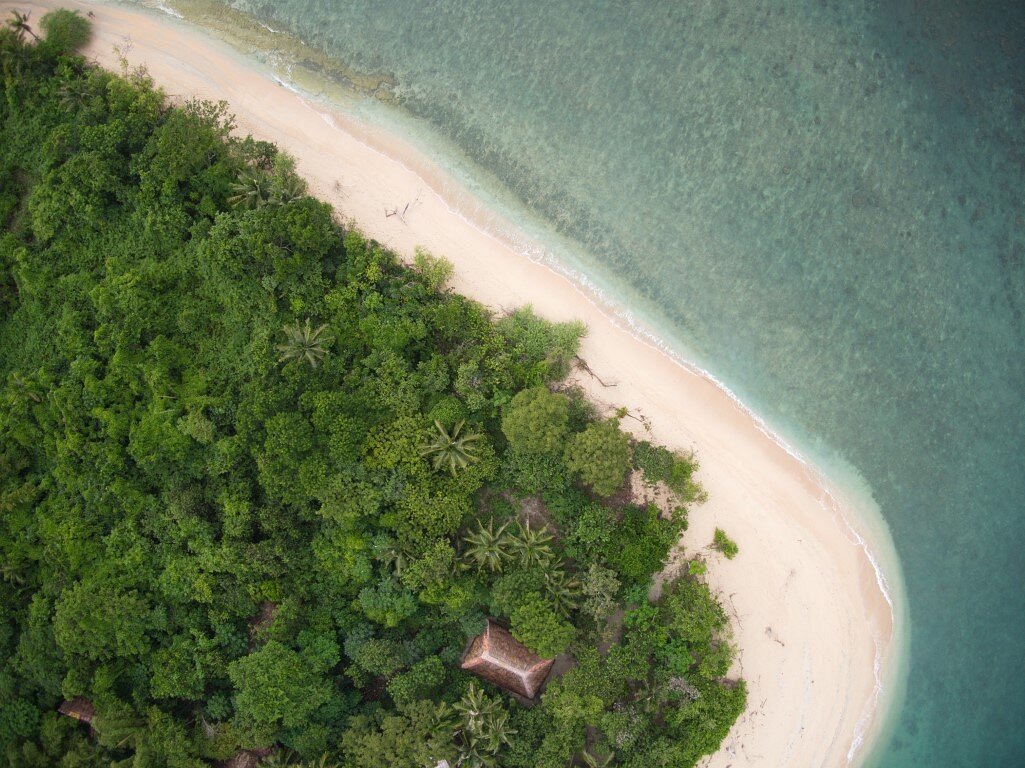This aerial photograph captures a serene beach landscape dotted with lush green vegetation and surrounded by tranquil ocean waters. To the left of the image, a dense cluster of trees forms a rich, green contrast against the sandy shore, which spans diagonally from the bottom center to the top right. The sand itself is a beautiful beige hue, suggesting a deserted, unspoiled beach. In the bottom center of the picture, partially surrounded by trees, is a building with a distinctive brown sloping roof. The water, which occupies the top right part of the image, displays a calming blend of pale blue and greyish hues with gentle ripples, adding to the overall tranquility of the scene. The combination of the lush vegetation, peaceful ocean, and isolated beach creates a picturesque outdoor nature landscape.